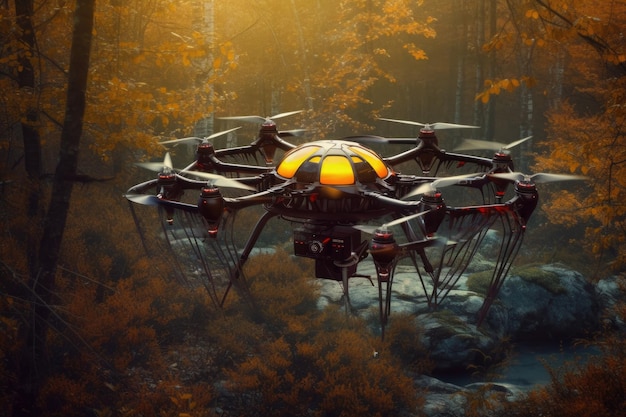The image depicts a large, futuristic drone situated in a dimly lit autumn forest. The forest is full of tall trees adorned with yellow and orange leaves, suggesting the season. The center of the image is dominated by the drone, which has a central circular body featuring an orange dome-like orb and six arms extending outward. Each arm is tipped with propellers, resembling helicopter blades, that are in motion as indicated by their blurry appearance. The drone is predominantly silver and red with white propellers and has parts extending downward from its base. It rests upon a bluish stone amidst a small rocky stream or pond, surrounded by scattered green patches, orange bushes, and dirt. Sun rays penetrate the canopy, casting a subtle glow on the scene, enhancing the drone's metallic sheen and the vibrant autumn foliage.